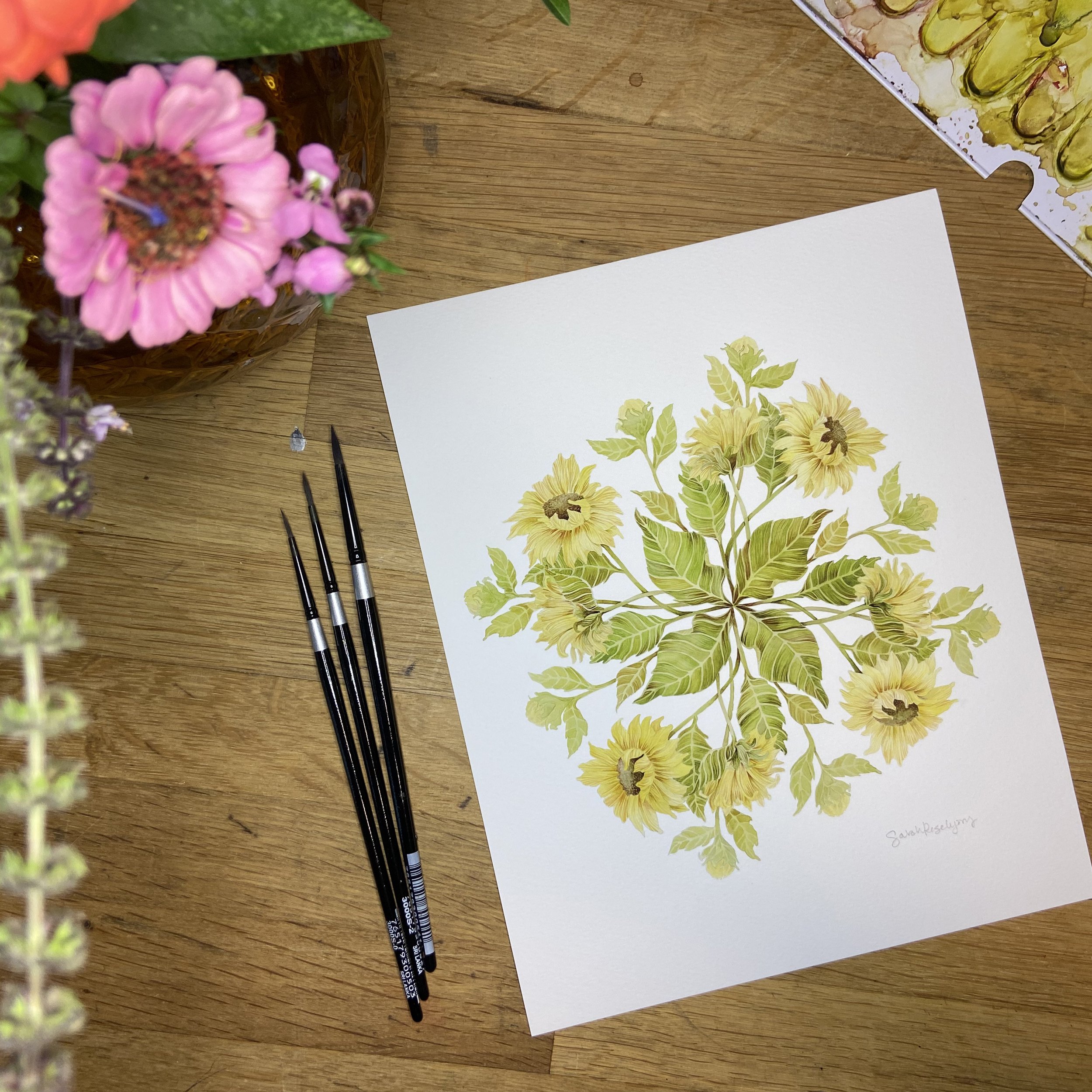The image features a meticulously detailed watercolor painting of flowers seen from an eagle's eye view on a plain wooden table. The composition showcases four light yellowish-green flowers, each situated in one of the corners—top right, bottom right, bottom left, and top left—curving slightly clockwise to form a pinwheel pattern. Interwoven among these blossoms, curling vines with slightly darker green leaves beautifully fill the spaces, enhancing the overall intricate design. 

Adjacent to the artwork, three thin paintbrushes with black handles and silver engravings are neatly placed, indicative of fine detailing. In the top left corner of the table, there is a potted plant with vivid pink petals surrounding a blue stamen, adding a splash of contrasting color to the setting. Another drawing is partially visible in the top right corner, although its details are indistinguishable. The artist's signature can be seen at the bottom right of the paper, albeit faint and difficult to read.

Overall, the intricacy and delicate color palette of the watercolor painting, combined with the surrounding artistic tools and complementary pink potted flower, create a harmonious and visually appealing scene, reminiscent of a potential book cover or card inlay design.